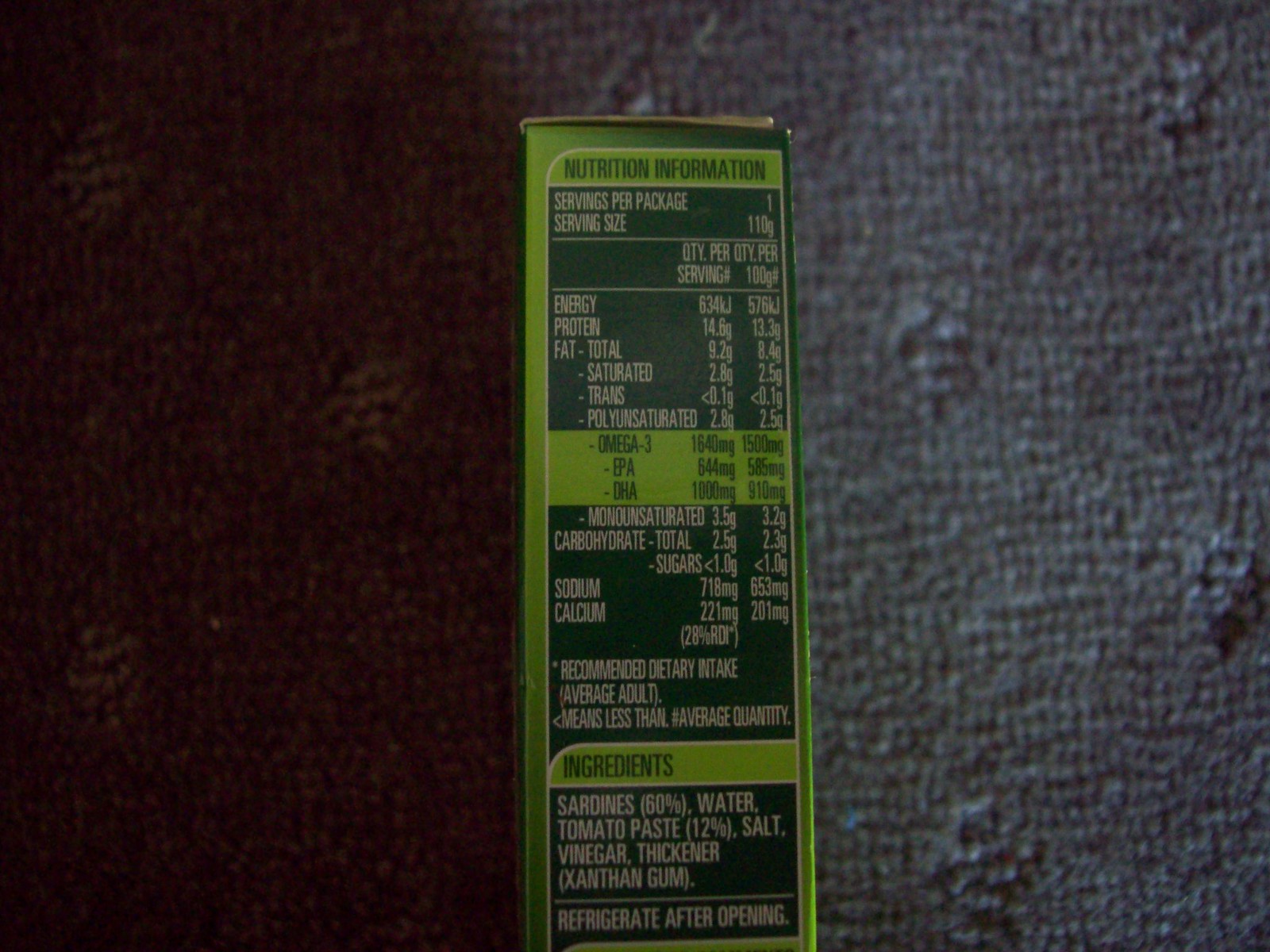The image is a close-up, albeit very dark, of the nutrition information on the side of a box, which appears to be positioned on a short carpet. The carpet is dual-toned; the left side is brown, while the right side is light gray and slightly illuminated, enhancing the gray's brightness. The box is orientated vertically, and the side panel features a dark green background with a lighter green trim. Most of the text is printed in white. 

At the top, the heading "Nutrition Information" is displayed against a potentially darker green background. Below this, it lists servings per package as one and the serving size as 110 grams. The section following, titled "Quantity per Serving," includes various nutritional details, though some numbers are difficult to discern. Categories listed under this section include energy, protein, fats (in total), saturated fats, trans fats, and polyunsaturated fats.

Further down, in a lighter green section, the text mentions omega-3 fatty acids, specifically EPA and DHA. The detailed numeric values are omitted due to readability issues.

Toward the bottom, the ingredients are listed as follows: sardines (60%), water, tomato paste, salt, vinegar, and thickener (XANTHAN gum). The instructions also advise refrigerating the product after opening.